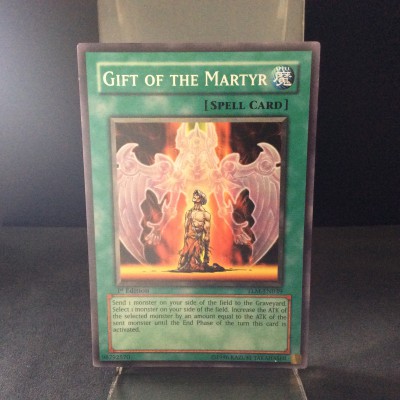The image features a prominently displayed playing card, set in portrait mode against a dark gray backdrop and resting on a matching gray table. This card, likely a magic or spell card, has a green background and is encased in a brown-bordered display with two small brown supports on the left and right sides. The top of the card reads "Gift of the Martyr" in bold text, and directly below, it is labeled as a "Spell Card" in parentheses. The central illustration depicts a shirtless individual seated in a chair, adorned with a red garment covering their lower half. Behind this figure, a semi-transparent, white crystal-like entity resembling a bat seems to hover, adding an aura of mysticism. Beneath the illustration, there is a brown-outlined text box containing approximately five lines of text, though the details within remain unreadable due to the zoom level of the image. The card appears positioned in a way that suggests it may either be part of a store display aiming to attract buyers or a personal collection piece showcased for admiration.